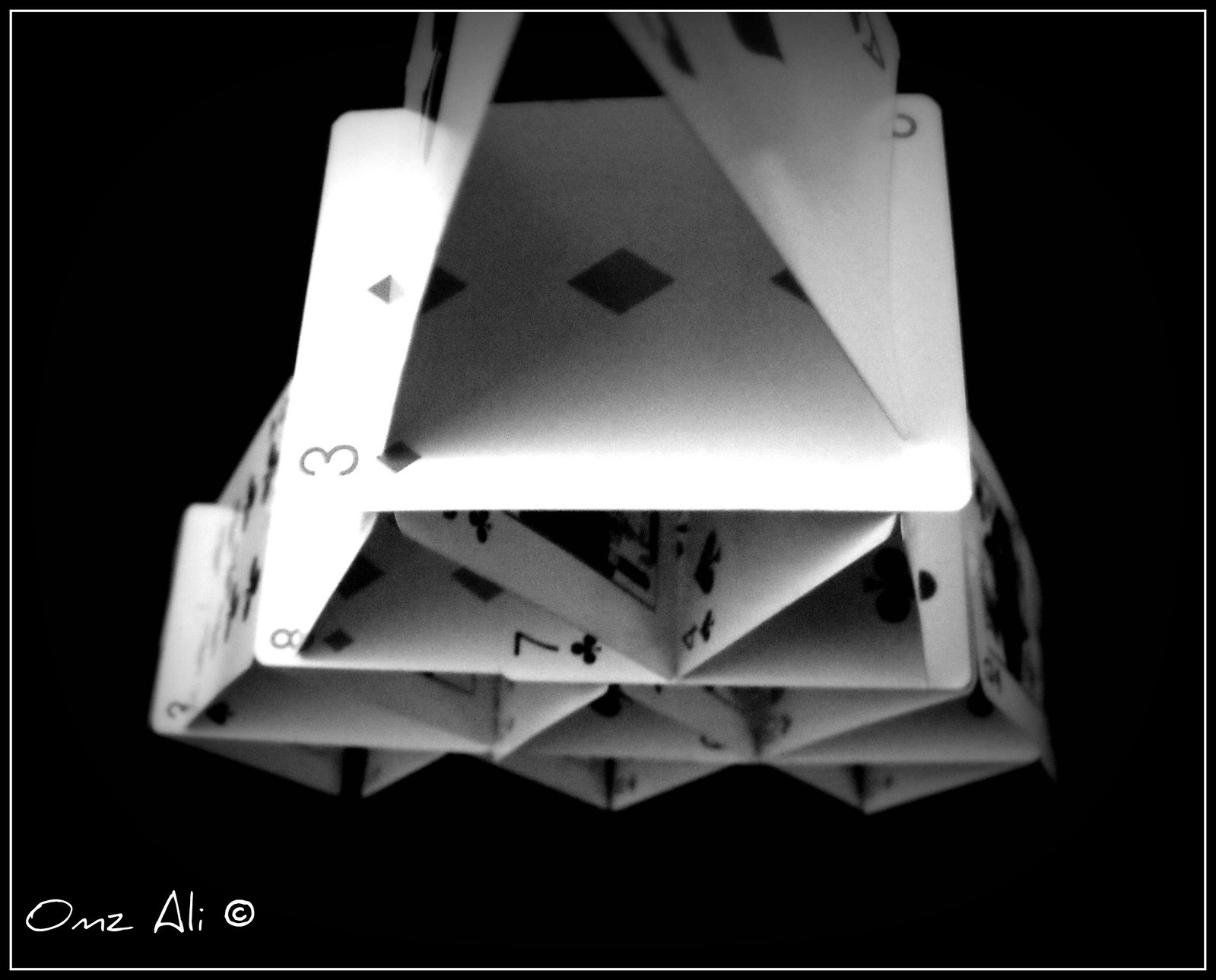The image features a meticulously constructed card tower, skillfully built using a portion of a deck of cards. The foundation starts with several cards placed diagonally, upon which three coherent rows of cards have been constructed. This structure further evolves into a fourth row, distinguished by cards artfully placed at varying angles on top of the third row to create a more intricate design. Noteworthy cards in the arrangement include the seven of clubs, three of spades, another unidentifiable card, and yet another seven of clubs, indicating the selective use of cards rather than an entire deck.

The backdrop of the scene is pure black, making the white cards vividly stand out in stark contrast. An inscription in the lower left-hand corner reads “OMZ Alley” with a circled 'C', possibly indicating the creator or the title of the piece. The image, captured from an overhead angle, offers a comprehensive view of the tower. One can appreciate the forward-facing sides and the complex, multi-dimensional arrangement, though the back of the tower is not visible. Overall, an estimated 16 cards have been used to bring this architectural marvel to life in an elegant and visually striking composition.